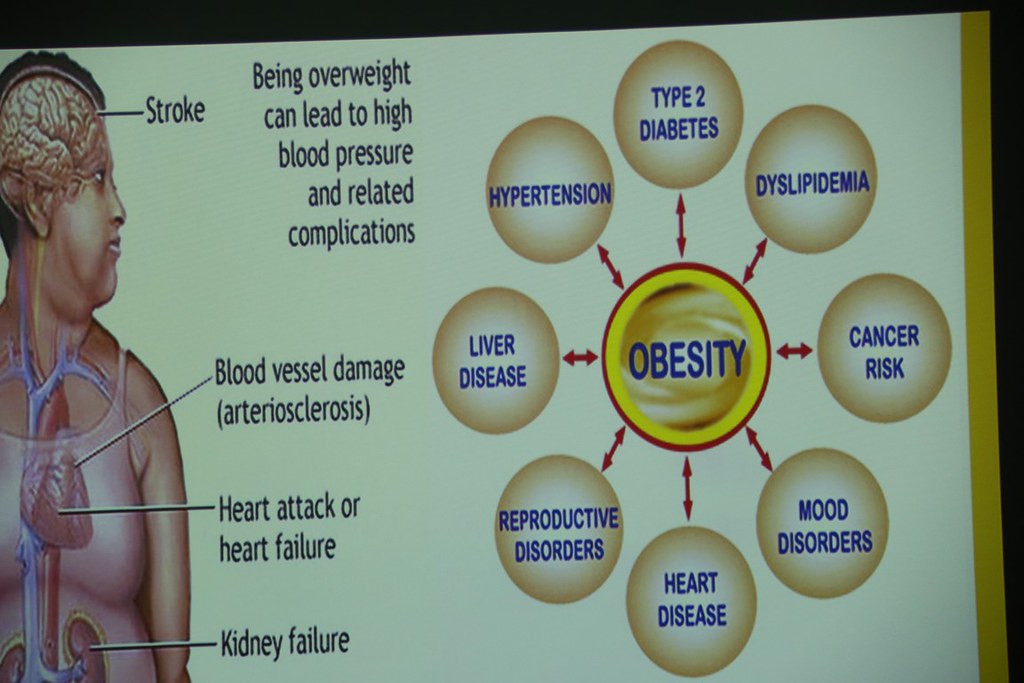The image is a close-up from a presentation slide with a slight background visible along the top and right edge. Dominating the left side of the slide is a cartoon sketch of a black woman seen in profile, revealing her internal organs—including the brain, heart, and kidneys. A black arrow points to her brain labeled "stroke," accompanied by the text "being overweight can lead to high blood pressure and related complications." Additional arrows indicate her heart with labels "blood vessel damage" and "heart attack or heart failure," while her kidneys are marked "kidney failure." Adjacent to this illustration, the right side features an infographic centered on the word "obesity" in bright blue letters encircled by yellow and red. This central bubble is interconnected with various white bubbles that denote conditions linked to obesity: "hypertension," "type 2 diabetes," "dyslipidemia," "cancer risk," "mood disorders," "heart disease," "reproductive disorders," and "liver disease," each marked with blue lettering and connected by red arrows.